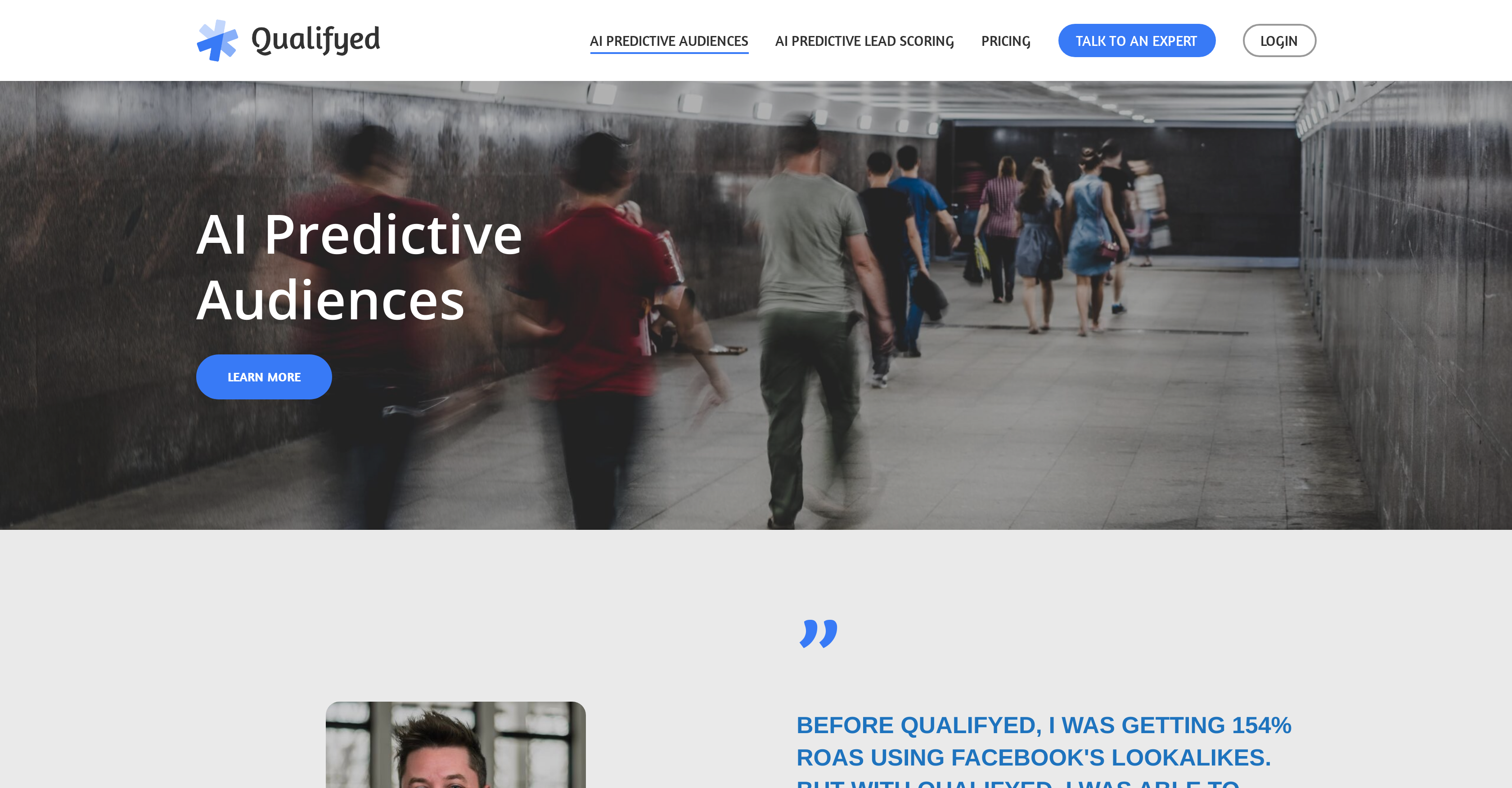This detailed caption for the screenshot describes the layout and elements of a website landing page for a company named Qualifyed:

"The screenshot captures the landing page of the Qualifyed website, featuring a logo in the top left corner comprised of crisscross lines forming a star, accompanied by the company name spelled 'Q-U-A-L-I-F-Y-E-D'. At the top, there is a navigation menu with clickable links labeled 'AI Predictive Audiences,' 'AI Predictive Lead Scoring,' 'Pricing,' 'Talk to an Expert,' and 'Log In.' The 'Talk to an Expert' button is highlighted in blue, and a line underscores the 'AI Predictive Audiences' link.

Directly below the navigation, a prominent section titled 'AI Predictive Audiences' displays an image of people walking through what appears to be an underground hallway. The scene suggests a subway tunnel, with a concrete block floor and smooth granite walls. Illuminating the space, lights are positioned along the top edges of the walls and down the center of the ceiling. The individuals in the image, both men and women, carry bags or jackets as they walk.

Beneath this 'AI Predictive Audiences' section is a 'Learn More' button. Scrolling further down, another section begins with a partially visible testimonial. Only the top of a man's head with dark brown or black hair is shown, alongside a partial quote reading: 'Before Qualifyed, I was getting 154% ROAs using Facebook lookalikes,' with the rest of the text cut off."